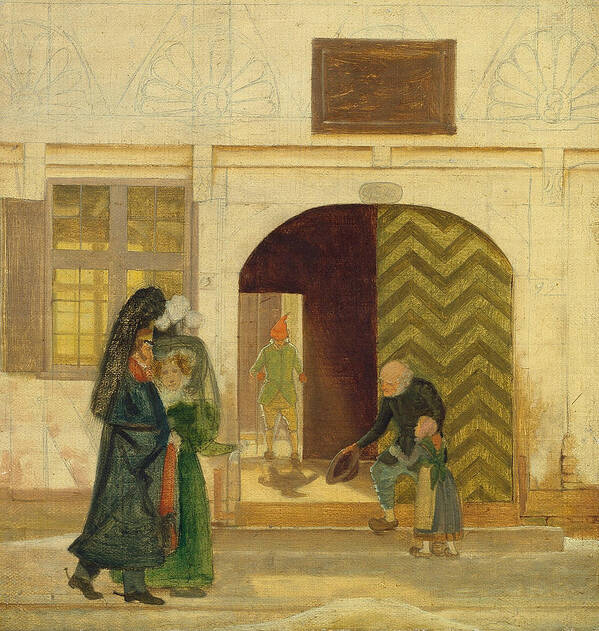This artwork is a vintage illustration featuring muted yellow tones and rich detail. The backdrop is a yellow-gold building characterized by a prominent archway entry in the center, above which lies a brown square. In front of this entryway stands an old man, bald, with a gray beard, wearing a dark coat and blue pants. He holds a brown hat in his right hand, and beside him is a young girl dressed in a blue gown with a white apron, her arms around her waist. Inside the archway, a man in a green jacket, beige trousers, and a red peaked cap can be seen walking out.

To the left of the archway stands a window, and nearby, a couple is seen walking together. The man, dressed in a floor-length black coat and a large headdress, sports a beard and sideburns. The woman at his side is adorned in an elegant full-length green dress and a grand hat with a green veil that drapes around her reddish-gold hair and fair skin. Her hat is embellished with three wide white feathers. The scene evokes a Victorian ambiance with its array of muted, vintage colors ranging from yellows and golds to greens and blacks.